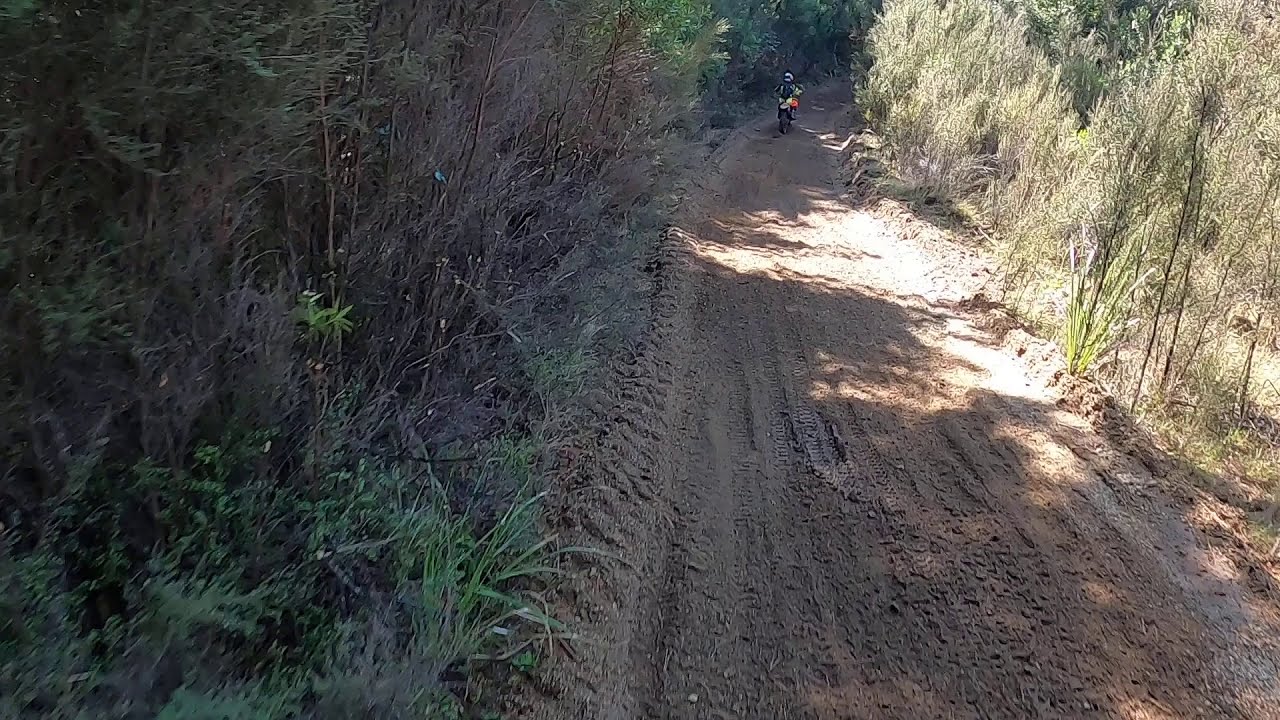The photograph features a wide, clay-colored dirt path coursing through a densely vegetated outdoor setting. The path, marked with numerous tire and tread impressions, extends from the foreground to a vanishing point in the upper right center, where it curves gently and becomes obscured by foliage. A single motorcyclist, tiny in the distance but slowly approaching, rides along this path. The rider, discernible by a helmet and indistinct dark clothing, has a conspicuous flash of red near their left hand on the bike.

On either side of the path, dense and somewhat dry vegetation thrives, including reeds, grasses, and varied brush in shades of gray, beige, and green. This lush undergrowth forms a natural canopy, allowing only sporadic sunlight patches to illuminate sections of the path, which appears brown and muddy in the shade and starkly white where touched by sunlight. The scene exudes a sense of seclusion, emphasizing the solitary rider's journey through this remote, sun-dappled woodland corridor.